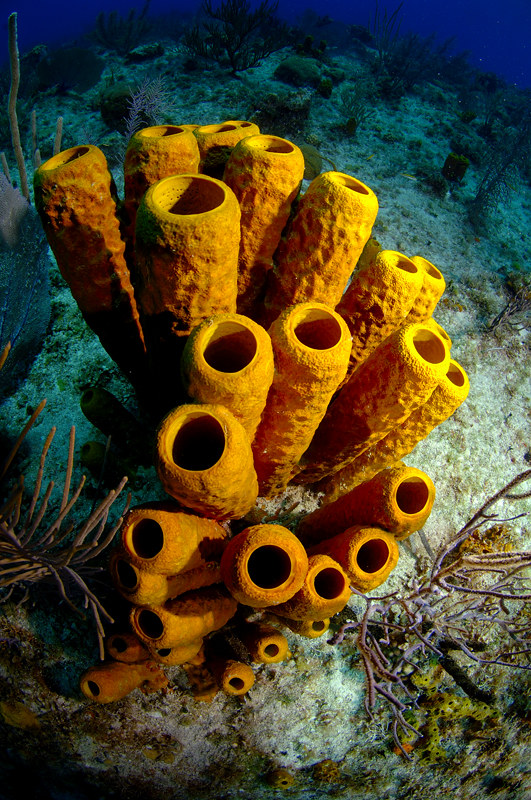This vibrant underwater photograph, taken in portrait mode, showcases a fascinating marine landscape. Central to the image is a large cluster of bright orange sea cucumbers, resembling rough, cylindrical tubes with open tops, each about two to three feet long. These tubular structures, around twenty in number, appear to grow together on a white seabed. Surrounding the sea cucumbers are various corals, including tree-like corals exhibiting a striking purple hue with intricate branch-like formations. The scene is set in shallow, clear turquoise waters, possibly around 15-20 feet deep, evoking the serene environment of the Caribbean. The background reveals turquoise and indigo shades of water, adding depth and contrast to the array of marine life, with scattered coral structures adorning the ocean floor.